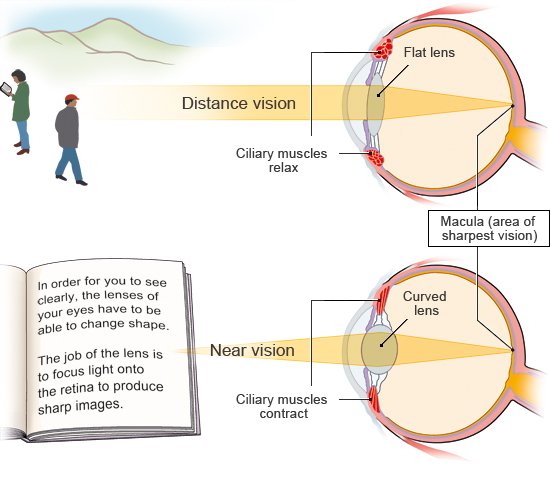This color cartoon-style diagram illustrates the differences between distant vision and near vision using side-by-side cross-sectional images of human eyes. The top right section of the diagram features the eye's anatomy labeled with the lens, different ciliary muscles, and the macula—designated as the "area of sharpest vision." Above this eye is a yellow arrow labeled "Distance Vision," which points to a scene showing a mountain with two people; one person is looking off into the distance while the other reads a book. The top eyeball is labeled "Flat Lens" and explains that the ciliary muscles relax for distant vision.

On the bottom right, another eye diagram is labeled "Curved Lens" for near vision, with a corresponding arrow indicating "Near Vision" pointing to an open book with text. This eye shows that the ciliary muscles contract to focus on nearby objects. The left section of the diagram holds a drawing of the book, with a quote: "In order for you to see clearly, the lenses of your eyes have to be able to change shape. The job of the lens is to focus light onto the retina to produce sharp images."

Overall, the diagram emphasizes how the eye accommodates vision at different distances by altering the shape of the lens, facilitated by the ciliary muscles.